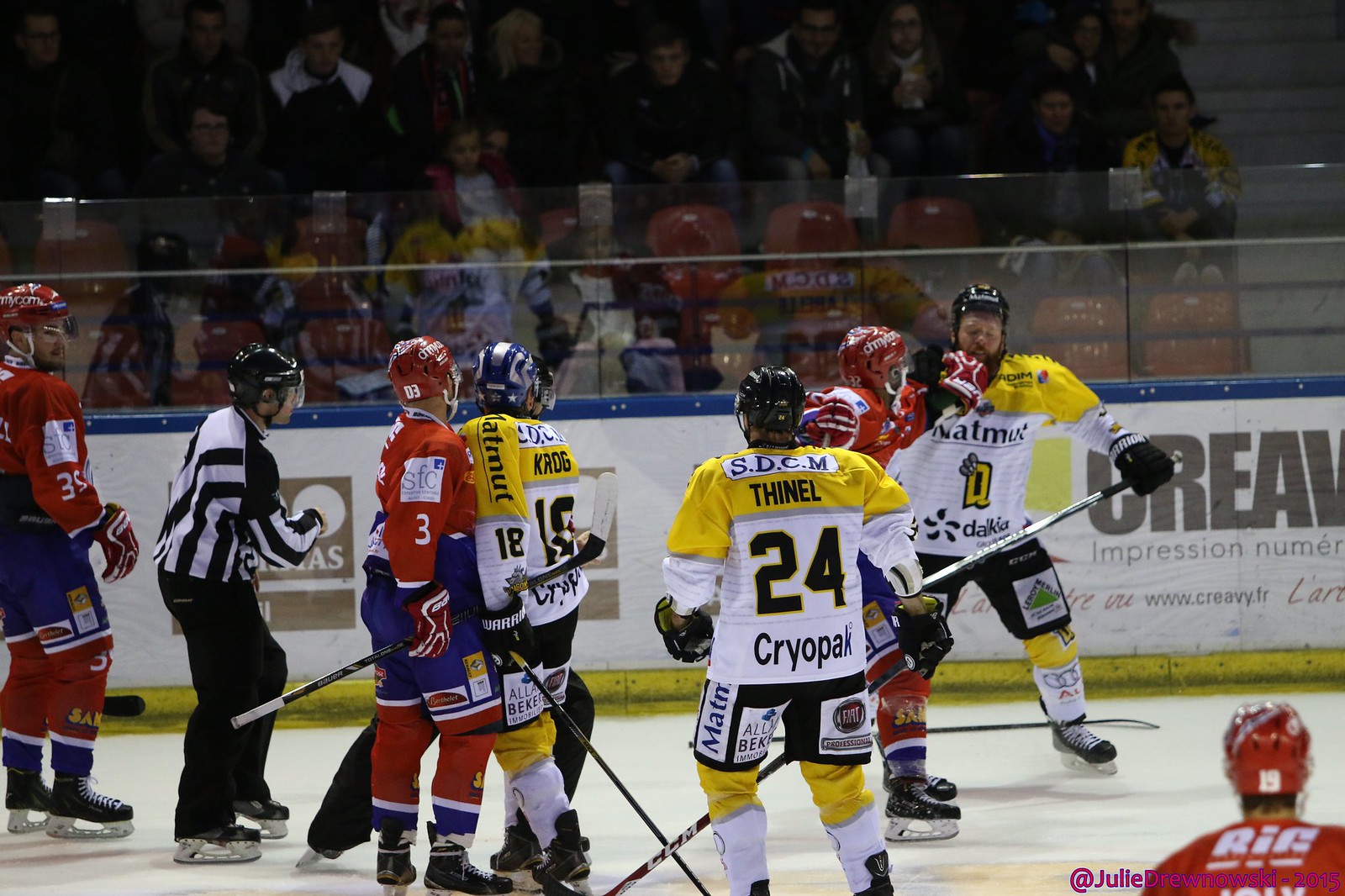The image captures an intense moment during a hockey game, frozen in time. Two teams are locked in a heated skirmish on the right side of the rink. The players, clad in contrasting uniforms, highlight the contest: one team features white and yellow jerseys with black shorts and numbers, while the other team sports red jerseys with blue shorts and red socks. Protective helmets and black skates are worn by all. At the center of the action, two players are engaged in a physical altercation, with a player from the red team seemingly punching a player from the white and yellow team. 

The referee, distinguishable in a black and white striped shirt and black pants, is moving in to intervene. Other players stand around, watching the confrontation. In the background, the transparent glass boundary of the rink offers a view of the audience seated in stadium-style bleachers, absorbed in the unfolding drama. The rink itself is encircled by a white wall featuring blue and yellow accents, and sponsor advertisements are displayed at the bottom. The scene is rendered in detailed, photographic realism, capturing both the dynamic action on the ice and the engaged spectators around the rink.